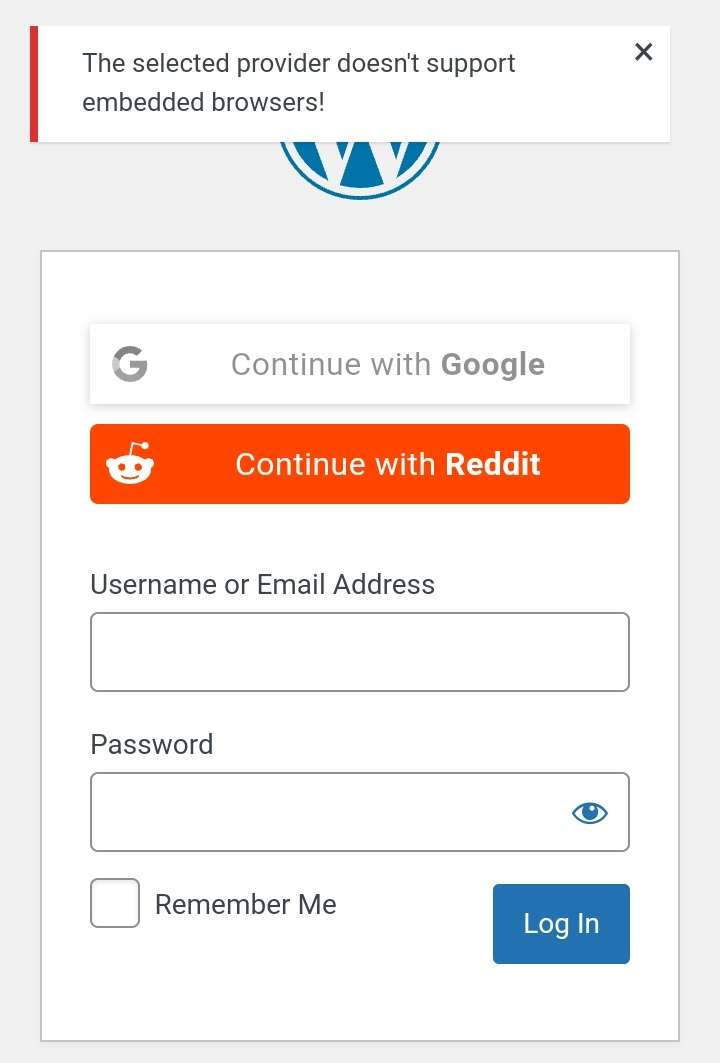A detailed descriptive caption for the image could be:

"This screenshot features a login interface set against a gray background. Prominently displayed is a red vertical line to the left of an error message stating, 'This provider doesn't support embedded browsers,' accompanied by a red 'X' icon. There is also a large blue circle containing a white 'W', which likely represents a specific platform or service. Below this, there are two distinct rectangular buttons: one orange with the bold text 'Continue with Reddit,' and another white button with bold text 'Continue with Google.' Beneath these buttons are individual input fields for 'Username or email address' and 'Password,' each depicted as rectangular boxes. A blue eye icon is positioned to the right of the password field, indicating a feature to toggle password visibility. To the left is a 'Remember me' checkbox. At the bottom of the interface, there is a prominent blue rectangle containing the word 'Log in' in white text."